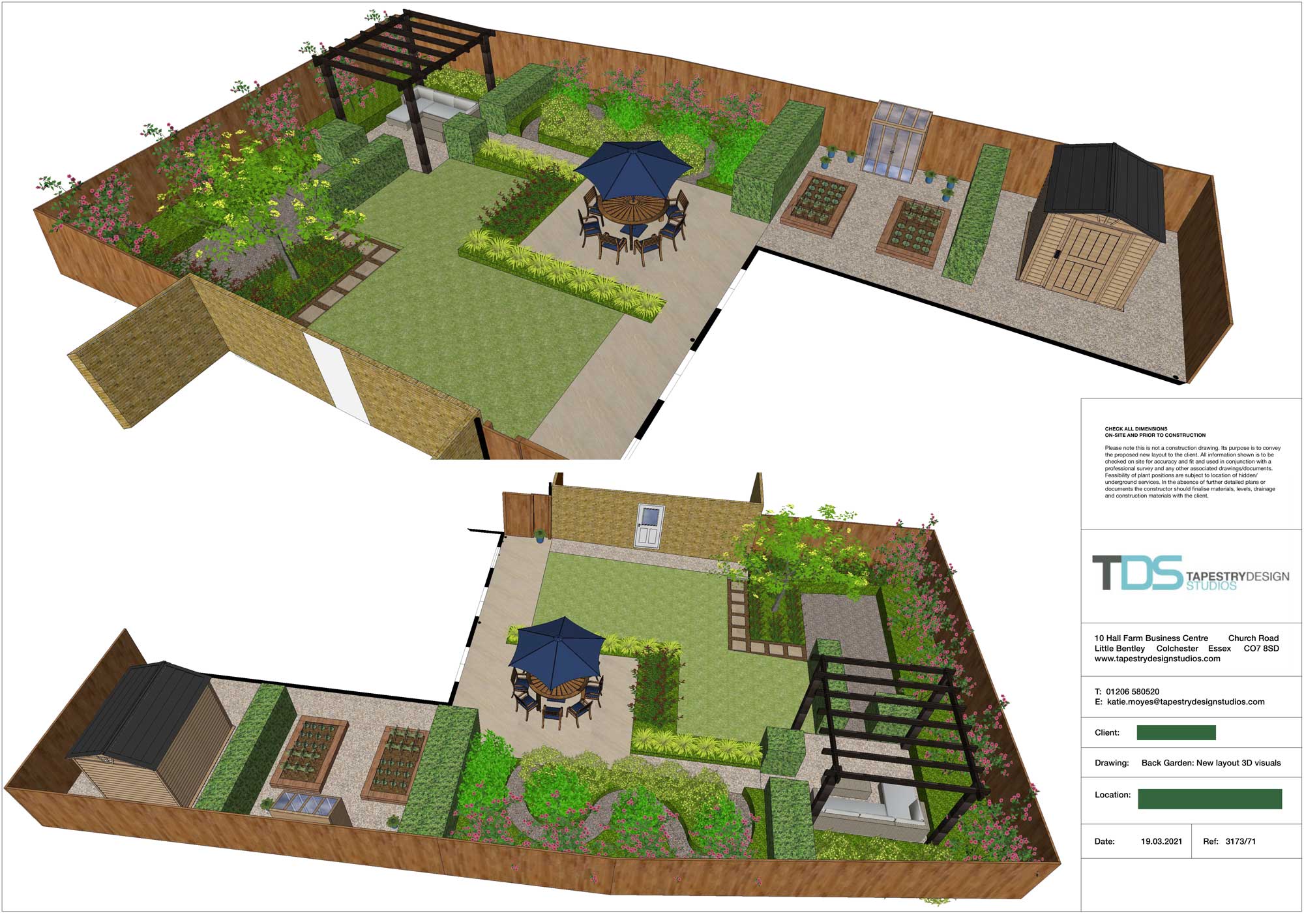This digital illustration created by Tapestry Design Studios showcases an intricate 3D representation of a landscaped outdoor garden, designed using advanced software modeling. The image clearly depicts a fenced-in backyard viewed from multiple angles, providing a realistic preview of potential garden arrangements. In the upper section, a shed is positioned on the right side, flanked by smaller garden beds to the left, and a larger square flower bed featuring a trellis in the upper left corner. Green grass areas are interspersed with cement walkways leading to various garden sections. A patio area is depicted with a table, blue umbrella, and surrounding chairs, enhancing the garden's recreational space. The bottom portion of the design presents an alternate view, rotated approximately 180 degrees, emphasizing different aspects of the layout. Additional features include a little gazebo and detailed information sections, although the text remains unreadable. The overall visual has a cartoony aesthetic, yet it allows homeowners to envision their ideal backyard layout vividly.